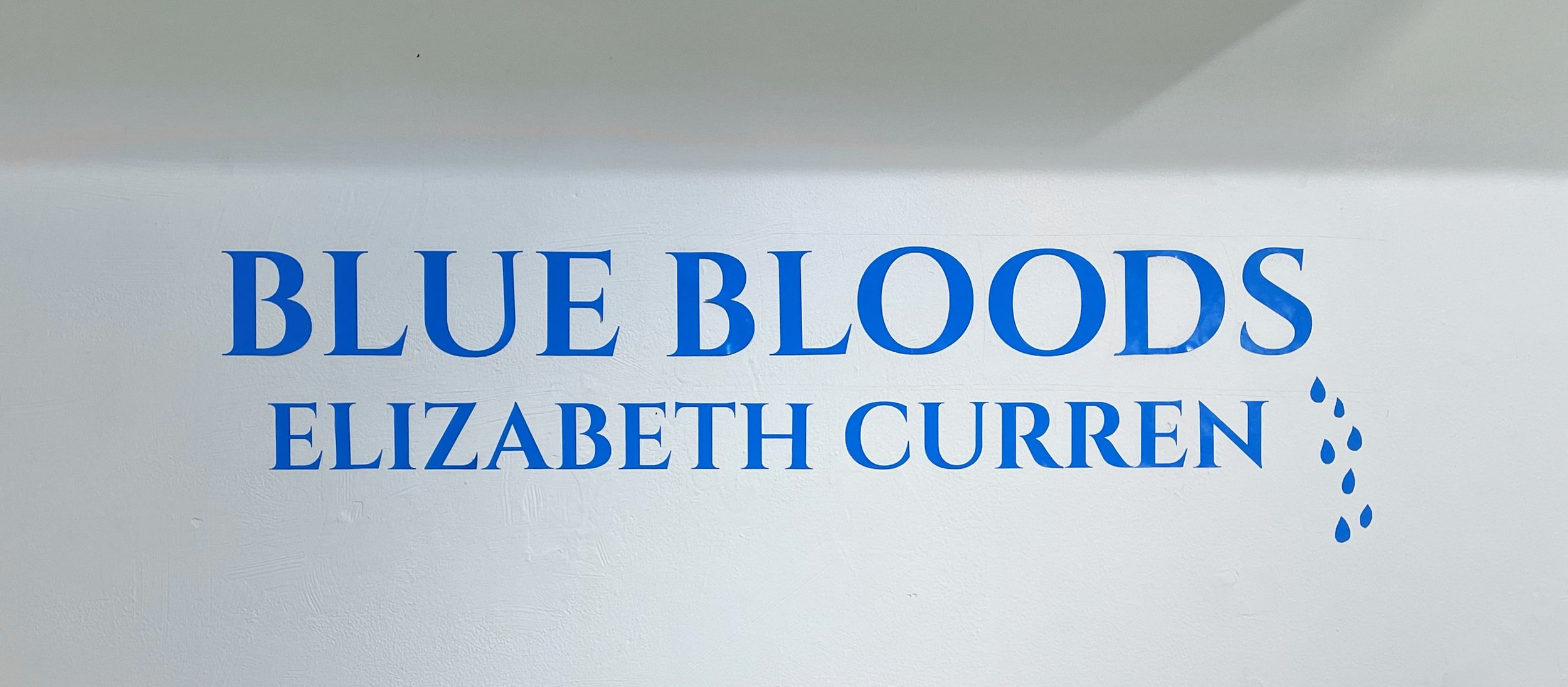The image is a rectangular advertisement, approximately 5 inches wide and 2 to 3 inches high. The background features a gradient of gray tones, starting darker at the top and gradually lightening towards the bottom. This gray background, which transitions to a nearly white hue, occupies the top quarter of the image before fading. The background also takes on a subtle bluish tint in certain areas behind the text. In the center of the image, there are two lines of blue serif font text. The first line, written in all caps and larger font, reads "BLUE BLOODS." Beneath this, in slightly smaller text but the same font style, it reads "Elizabeth Curran," with the spelling C-U-R-R-E-N. From the 'S' in "Blue Bloods," blue droplets resembling water or blood drips extend downwards towards the right side of the image, adding a distinctive design element to the composition.